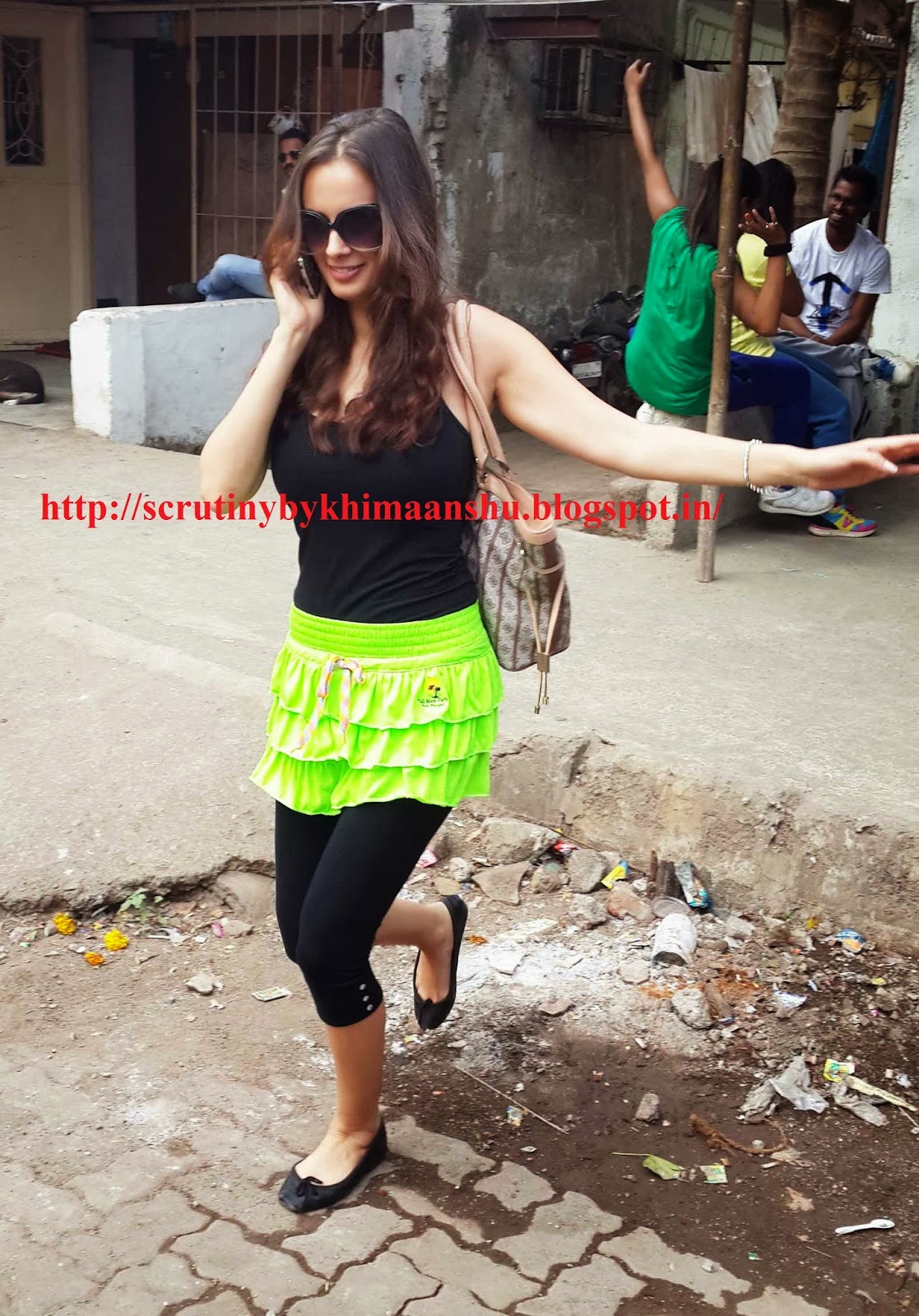The image captures a lively yet rough outdoor street scene, seemingly set in an economically disadvantaged area possibly in a foreign country. The backdrop reveals weathered concrete walls with clothes hanging on lines and metal bars framing a doorway, reflecting a sense of hardship. Scattered debris litters the ground, further emphasizing the area's dilapidated state.

In the background, four individuals are visible: two women and two men. One man, positioned on the left, wears sunglasses and sits on a concrete structure, gazing towards the camera. The other three individuals are engaged in a cheerful conversation, their expressions filled with laughter. Despite the grim surroundings, their interaction adds a touch of warmth to the scene.

Dominating the foreground is a stylish woman with long, curly brown hair, donning sunglasses, a black tank top, a bright green skirt with black leggings, and black ballet shoes. A purse hangs over her left shoulder. With one hand raised and the other holding a phone, she appears to be dancing and enjoying herself, exuding happiness and energy. The vibrancy of her attire and demeanor starkly contrasts with the surrounding poverty.

Across the lower section of the image, red text reads, "scrutiny by kimanshu.blogspot.in," suggesting a commentary or critical observation by a blogger named Kimanshu.